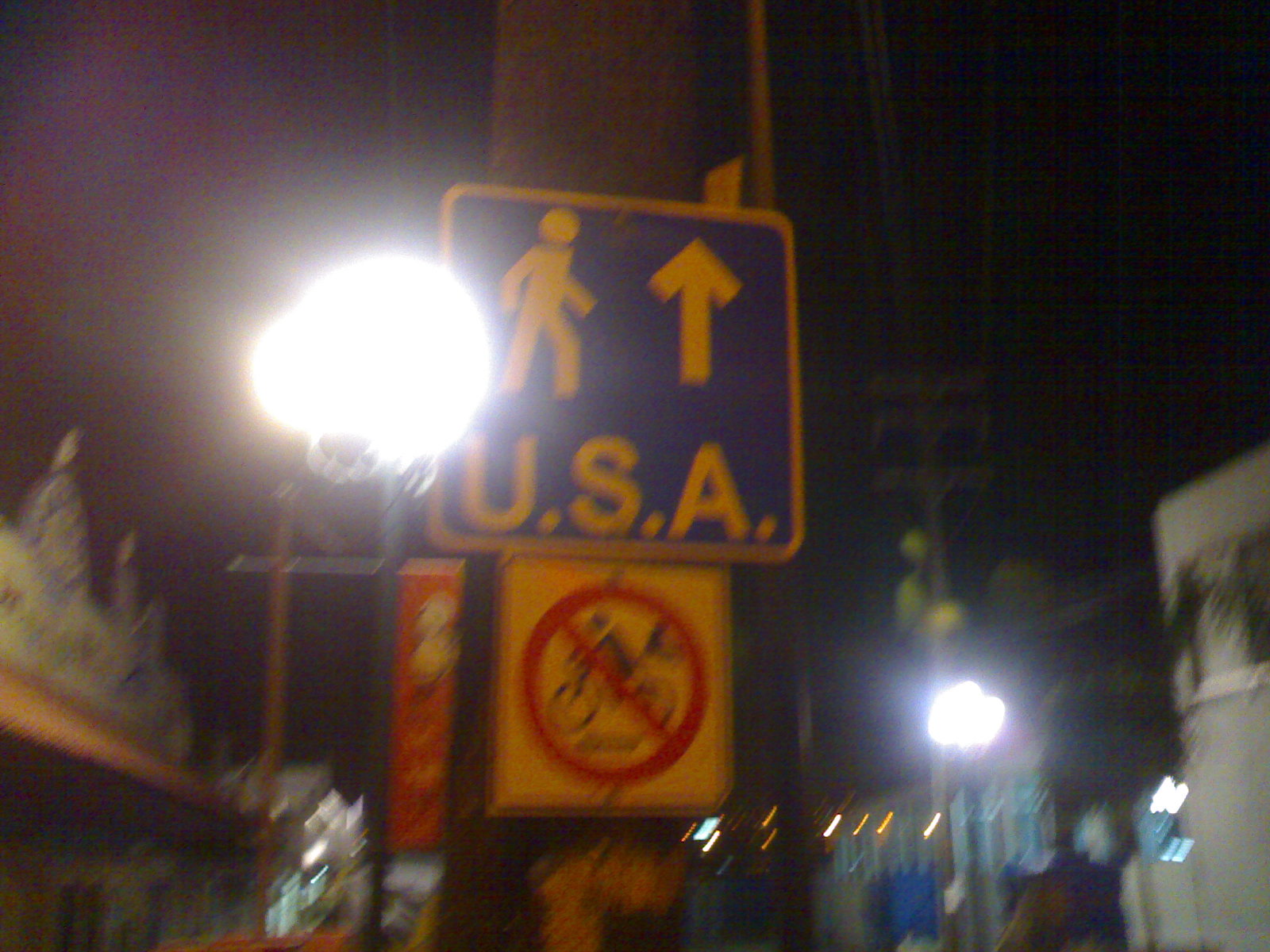In the nighttime image, we are gazing upwards at two prominent signs against a dark sky with a faded purple hue in the top-left corner. The lower sign is a yellow square featuring a black silhouette of a person on a bicycle, encircled in red with a diagonal line crossing through it, indicating that cycling is prohibited. Above it, a square blue sign with an orange border displays an orange stick figure, a rightward arrow, and the word "U.S.A." also in orange. To the left and right of these signs are bright beams of light, casting an eerie glow. The image also showcases blurry outlines of building structures, tree leaves, and a telephone pole in the background on the right.